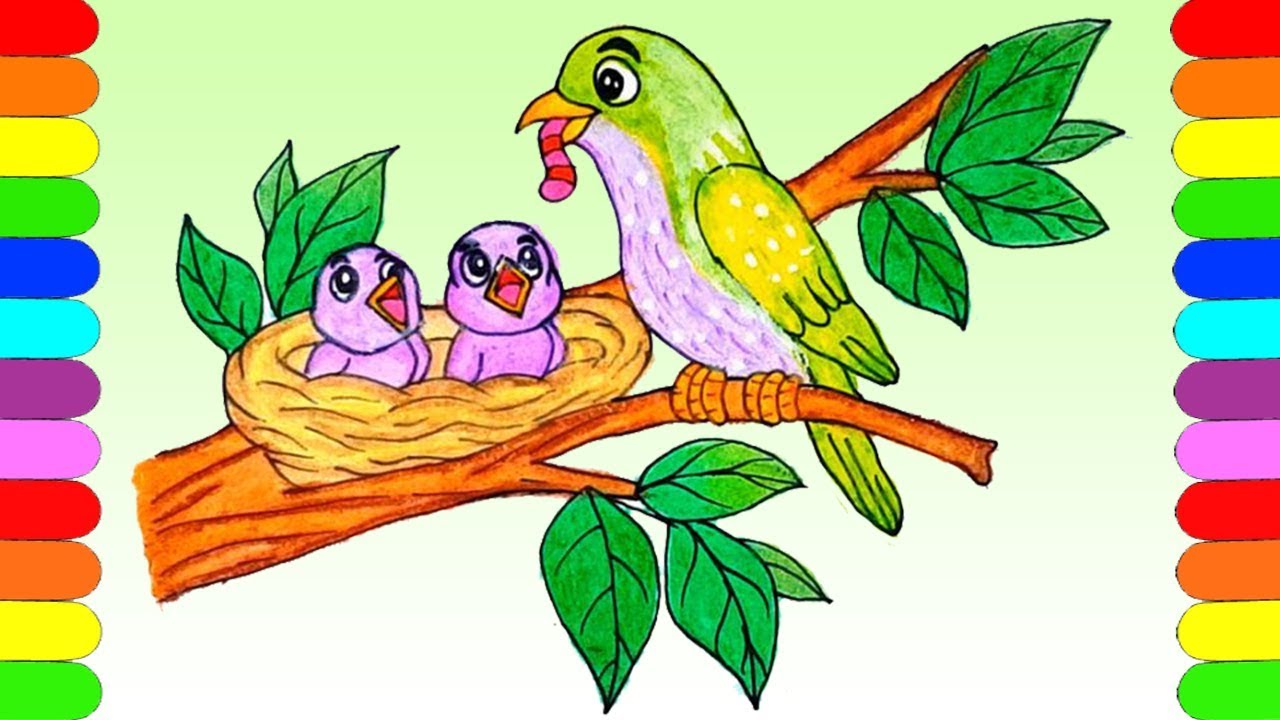The image is a vivid and colorful, kid-friendly illustration, resembling a scene from a children's book. At the center is a charming depiction of a green mother bird, with a yellow-tipped wing and a purple chest extending from its neck down to its legs. The bird, perched on a brown branch extending diagonally from the bottom left to the top right of the frame, holds a pink and red striped worm in its beak. The mother bird features distinct white eyes with black pupils and a black eyebrow, adding to its expressive look.

Below, in a carefully crafted brown nest with wavy twig details, sit two baby birds with purple feathers and yellow beaks. These chicks, eagerly looking up at their mother, have their mouths wide open in anticipation, displaying the pink interior of their mouths. Like their mother, they also have black eyebrows, lending them a similar look of curiosity and eagerness.

The surrounding scene is detailed with green leaves shaped like retro Christmas lights, complete with black veins, giving a vivid and playful touch to the foliage. Framing the image on both the left and right sides are vertical sequences of rainbow-colored, curved-top rectangular tabs. These tabs repeat in the order of red, orange, yellow, green, dark blue, light blue, dark purple, light purple, and then repeat once more, adding a whimsical border to the composition. The background transitions from a light green gradient at the top to white at the bottom, enhancing the overall cheerful and inviting aesthetic of the illustration.